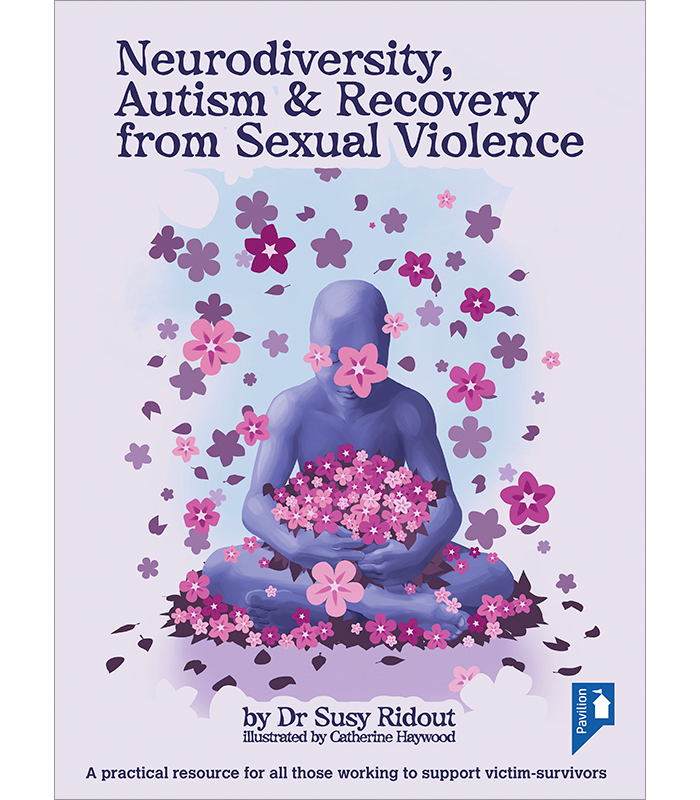The image is a detailed graphical poster with a light violet background, prominently titled "Neurodiversity, Autism, and Recovery from Sexual Violence" in black text at the top. Below the title, there is a watercolor illustration of a bald human figure with blue-shaded skin, sitting cross-legged on the ground with closed eyes. The figure is depicted holding a large bouquet of flowers in shades of pink, purple, and white, with additional flowers falling from the sky and scattered around its body on the floor. At the bottom of the image, there is black text reading "By Dr. Susie Ridout, Illustrated by Katherine Haywood," along with the phrase "A practical resource for all those working to support victim survivors." On the bottom right corner, there is a blue and white logo with the text "Pavilion."